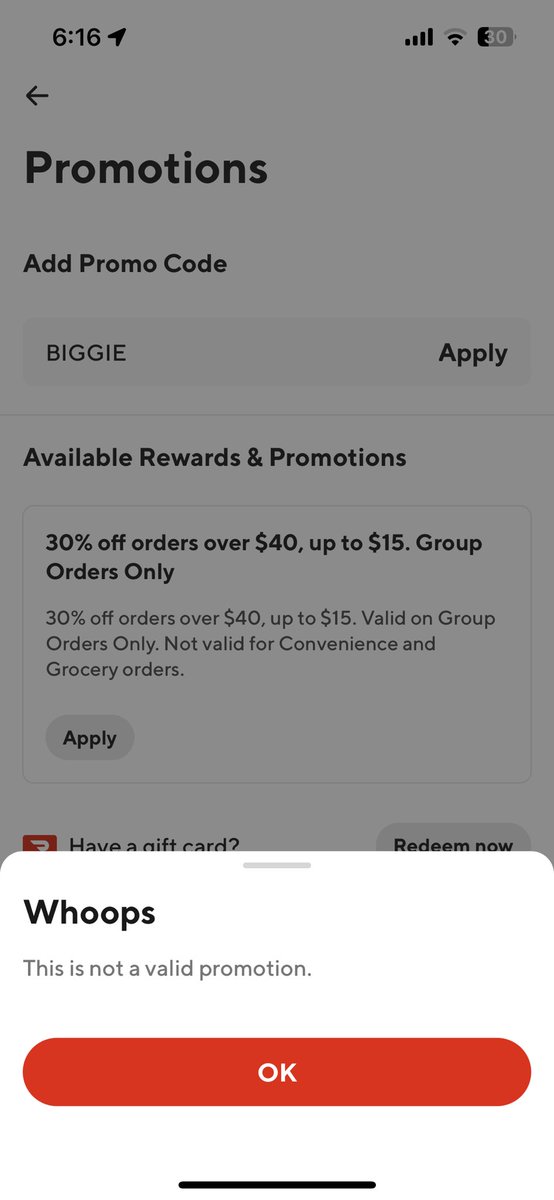The screenshot displays a detailed interface of a mobile application. At the top, within a gray box, is "616" indicating possibly the time, and next to it, it shows the battery level at 30% and a signal strength of four bars. An arrow pointing left, likely a back button, is also visible. The screen prominently features text displaying "Promotions" and an entry field labeled "Add Promo Code." 

Below this is a box containing the word "Biggie" spelled as B-I-G-G-I-E with an "Apply" button adjacent to it. Underneath this section, a horizontal line spans from left to right, demarcating the area from the subsequent section titled "Available Rewards and Promotions."

In this section, there's a box providing details of a specific promotion: "30% off orders over $40, up to $15, group orders only." The description emphasizes that this discount is valid only on group orders and excludes convenience and grocery orders. Next to this promotional box are two buttons labeled "Apply" and "Redeem Now."

Further down, there is a message, "Whoops, this is not a valid promotion," accompanied by a red "Okay" button beneath it. Lastly, a black horizontal line spans the width of the screen below this notification.